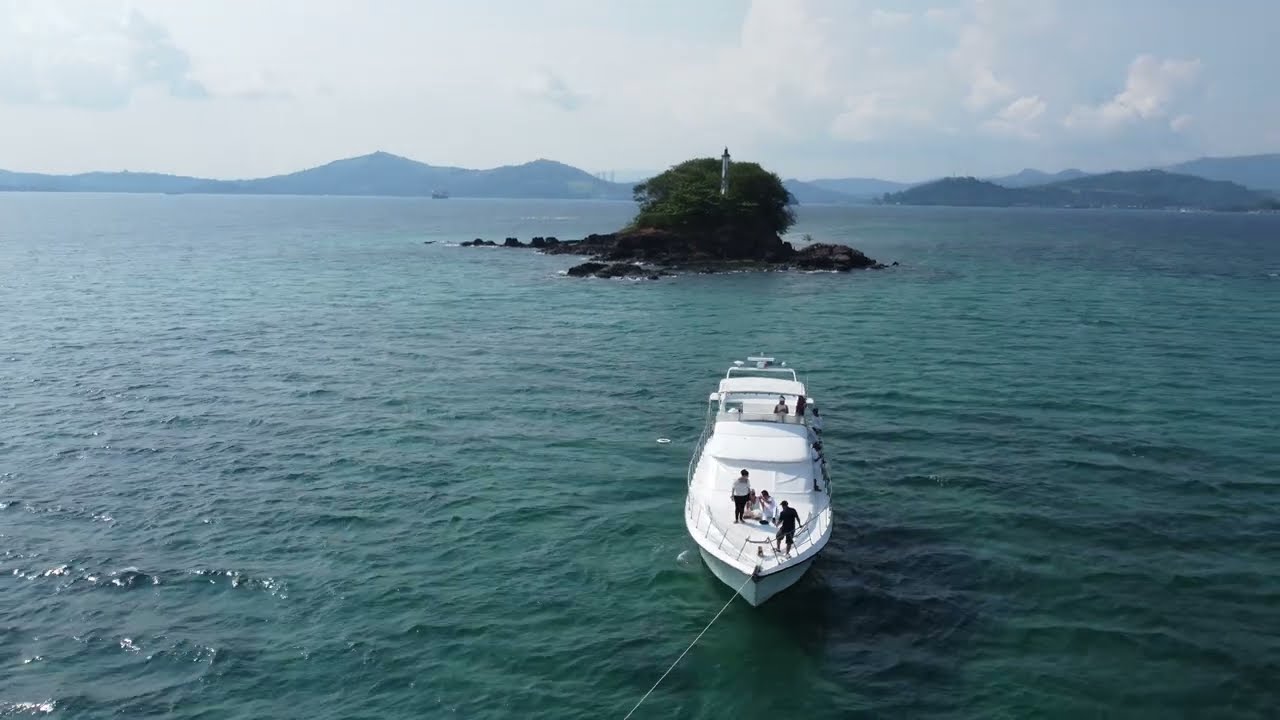The image depicts a picturesque scene of a large body of water, possibly a lake or an inlet from the sea, occupying the bottom 75% of the frame. The water appears in varying hues of aqua, dark blue, and even almost black due to the lighting. Prominently featured in the foreground is a wide, white boat with its bow facing the viewer. At least four people are visible on the boat: three towards the front and one positioned where the steering wheel would be, suggesting the boat is not moving and possibly anchored by a rope extending from its bow off to the left.

In the middle distance is a small grassy island adorned with green trees. At the center of this island stands a vertical, cone-shaped man-made structure, which could resemble a lighthouse or similar building. The island is bordered by rocks, adding to its rustic charm.

Further back, the background reveals undulating hills under a partly cloudy sky that appears bright blue despite the presence of clouds. In the far distance, there might be a bridge partially visible, along with a small speck that seems to be another boat on the water. The scene is a blend of natural and man-made beauty, capturing hues of white, green, and blue harmoniously.